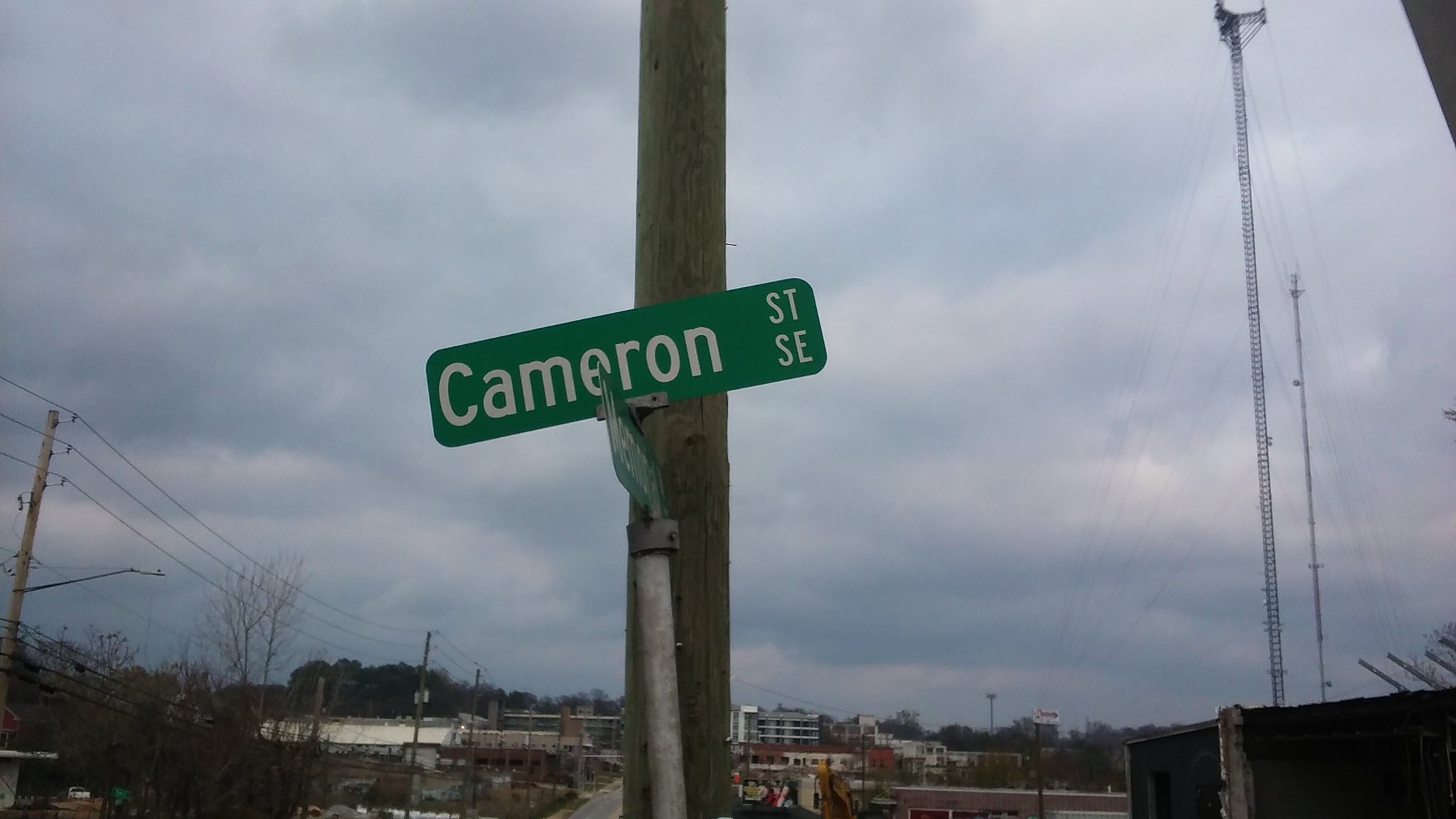This color photograph, taken outdoors in landscape mode, features a detailed street scene dominated by a series of structures and atmospheric conditions. Central to the image is a grey pole that runs vertically from top to bottom, with a green rectangular street sign attached to it, bearing white lettering that reads "Cameron ST SE". Surrounding this sign, the sky occupies around 90% of the photograph and is filled with dense grey and white clouds, suggesting an imminent rainstorm. 

A large wooden telephone pole, clamped to which is the grey pole, is also visible. To the bottom left, several power lines stretch diagonally, while towards the right edge, there is a tall structure, possibly a communications tower, with wire cables forming an inverted V-shape at its top. Beneath it, a smaller electrical tower stands. Additional details include the faint landscape at the bottom of the image, where trees—some bare—and distant buildings of various sizes are silhouetted. Furthermore, a black shadow appears in the bottom right-hand corner, and a black triangle is present in the upper right-hand corner.